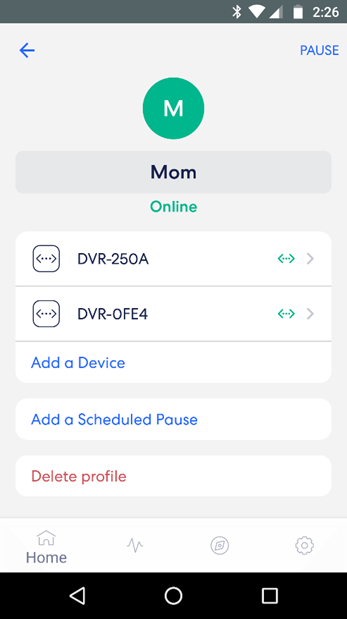This is a detailed screenshot from a mobile phone interface. At the top of the screen is a gray status bar displaying various icons in white font. On the upper right, there are icons for Bluetooth, Wi-Fi, mobile signal, battery status, and the time, which reads 2:26. Directly beneath the status bar, the main part of the interface appears to be an open settings menu against a gray background.

In the upper left corner of the settings menu is a small blue arrow pointing to the left, typically indicating a "go back" action. In the upper right corner, "Pause" is written in blue font. Centrally positioned is a darker gray circle containing a white letter 'M'. Below this circle is a gray rectangle with "Mom" written in black font, along with a status indicator reading "online."

Further down, there are two white rectangles. The first one reads "DVR-250A" and the one directly below it reads "DVR-OFE4." Continuing down, another white rectangle with blue font says "Add a device." Beneath this, yet another white rectangle with blue font states "Add a scheduled pause." Finally, at the bottom of this part of the interface, there is a white rectangle with red font stating "Delete profile."

At the very bottom of the screen is a navigation bar with a white background, featuring four icons. The first icon is a house symbol, with the label "Home" directly below it.